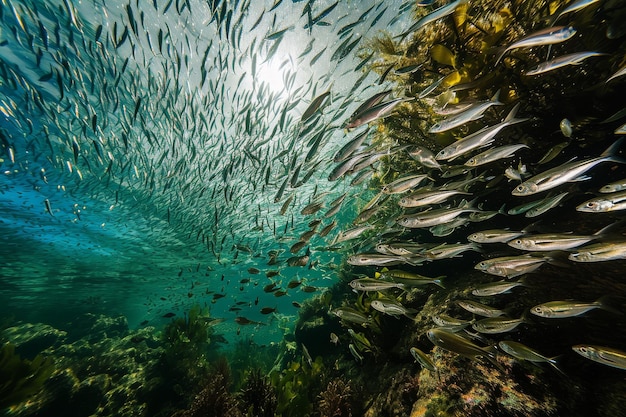The image captures an enchanting underwater scene with a large school of slender, silver fish adorned with black lines along their bodies. These fish appear to number in the hundreds, swimming in a coordinated, almost tunnel-like formation. The water is a striking teal-green, particularly vivid in the upper right corner where you can see a clear outline of this vast school. The reflection of the sun forms a small white spot at the upper center, casting a luminous glow over the scene. 

In the foreground, the bottom left showcases verdant underwater plants, while the right side features a rocky shelf covered in what appears to be green algae with some yellowish leaves. The clarity of the water allows for detailed viewing of the fish in this area. The background and the fish above the right shelf create a dense mosaic of life, emphasizing the richness and depth of the underwater world.